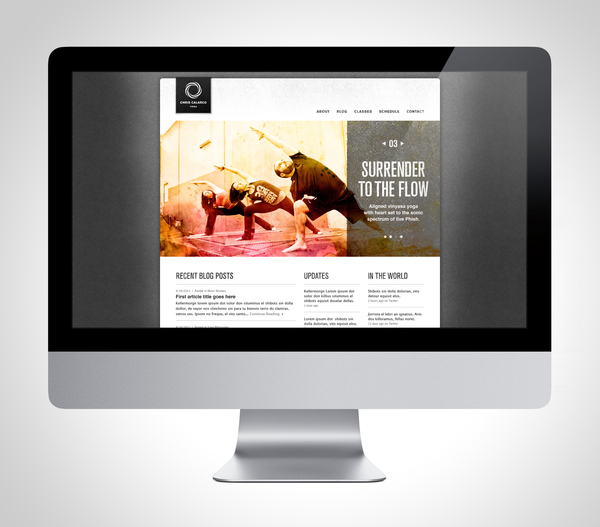The image depicts a screenshot of a computer monitor, likely an Apple device, distinguished by its sleek silver stand and matching silver bottom bezel, although it lacks the prominent Apple logo. The screen itself features a black bezel. 

Displayed on the monitor is a web page dedicated to yoga. Central to the web page is a stylized illustration of three individuals striking a yoga pose, their arms elegantly stretched out as they bend to their left. To the right of this image, clear text reads "03 Surrender to the Flow."

A menu bar runs along the top right section of the screen, though the text is too small to decipher clearly. Notably, the last menu item, situated close to the right edge, appears to be "Contact."

Above the main yoga image, on the left side, is the company logo. This logo features a black background with a design resembling a circle formed by intricate white lines. Below the yoga illustration, the page is divided into three distinct columns. The leftmost column is labeled "Recent Blog Posts," the middle column is titled "Updates," and the rightmost column is named "In the World."